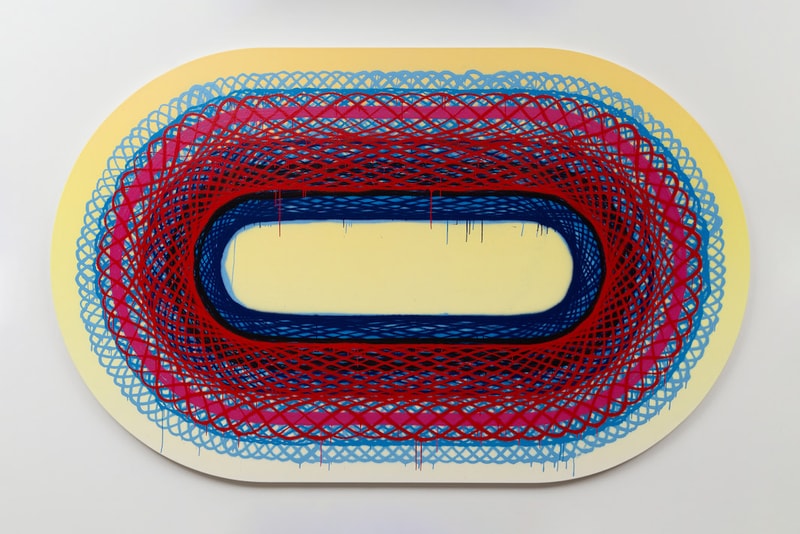The image features an ornate, oval-shaped design that resembles a woven carpet or intricate textile. The outer edge of this oval is bordered by a bright yellow band. Moving inward, the next layer consists of light blue with a spiral pattern woven into it. This is followed by a dark red or maroon layer featuring a cross pattern, also evoking a woven texture. Continuing inward, there is a more densely woven section with dark blue and a cross pattern. In the very center, the design concludes with a solid dark blue, still maintaining the woven appearance. 

The entire oval shape is positioned on a light green surface. Both the top and bottom edges of the oval bear small flags. Additionally, there are paint splotches, subtly dripping down from the top and bottom edges of the image, adding an artistic touch to the overall composition. The complex interplay of colors and patterns within the oval creates a visually striking and textured effect.